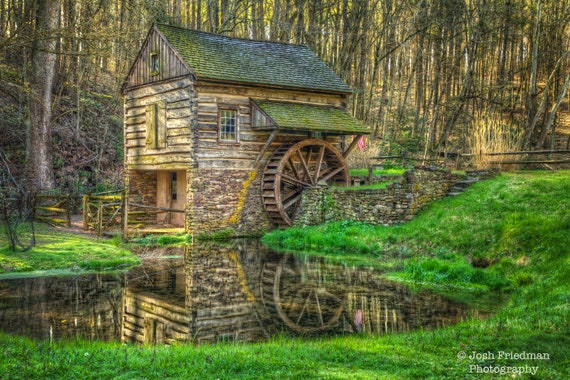This image depicts a charming rustic cabin nestled in a lush wooded area. The two-story structure has cream or brown walls, accented by a green triangular roof. A large wooden water wheel, likely used for generating electricity, is attached to one side of the cabin. The picturesque scene includes a serene pool of water in the foreground, which mirrors the cabin's reflection on its surface. Surrounding the water, lush green grass blankets the ground, and tall trees frame the background, enhancing the tranquility of the setting. The cabin features several windows, strategically placed on different sides, adding to its quaint and inviting appearance.